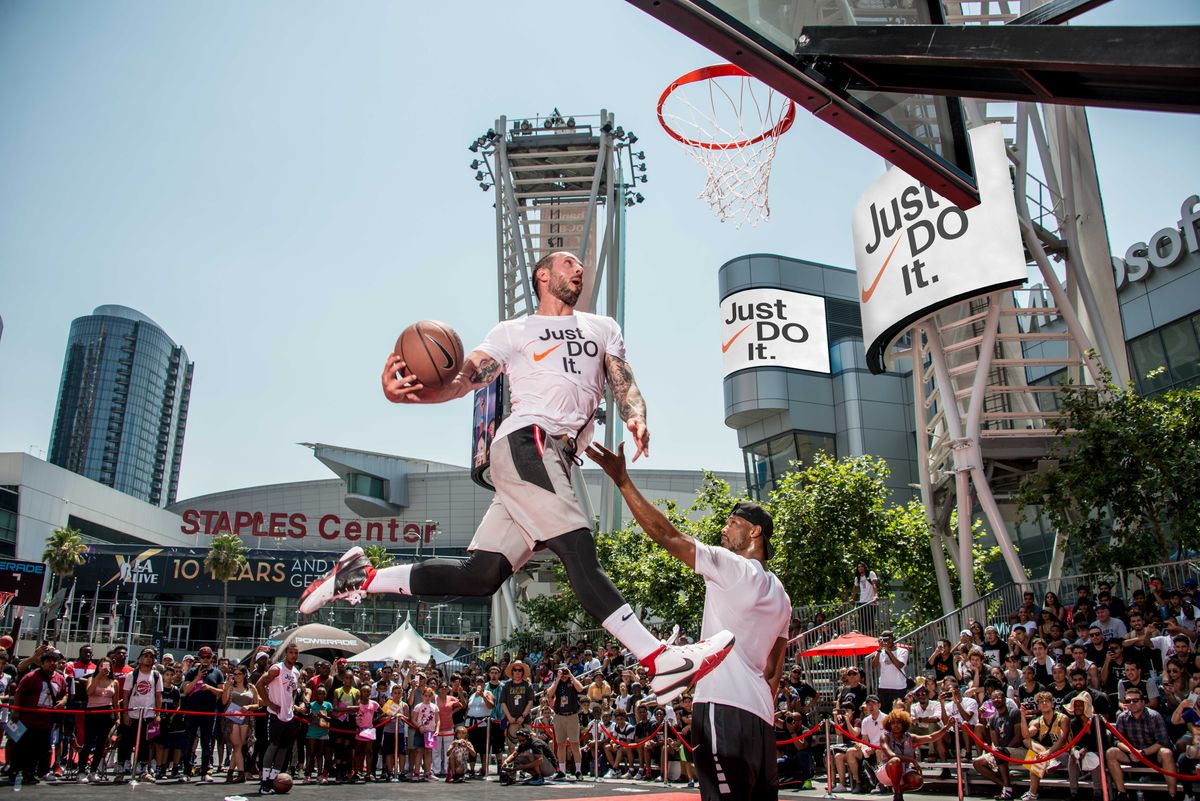The vividly detailed image captures an intense moment during an outdoor basketball game. At the center of the action is a man mid-air, poised for a powerful slam dunk. He dons a white t-shirt emblazoned with "Just Do It" in bold black letters beside a striking orange Nike logo. His outfit includes grey shorts and stylish black and white sneakers, complemented by white socks. The player's arms, adorned with tattoos, grip the basketball as he approaches the hoop. In close proximity, another man stands with his hand raised, seemingly attempting to thwart the impending dunk. This defender wears a white t-shirt and black shorts. The scene is set against a backdrop of a lively crowd gathered around the court, with the iconic Staples Center and various buildings, including one featuring a "Just Do It" sign, visible. Framed by a clear, bright blue sky, the image is bathed in natural light, showcasing impressive clarity and vibrant colors.